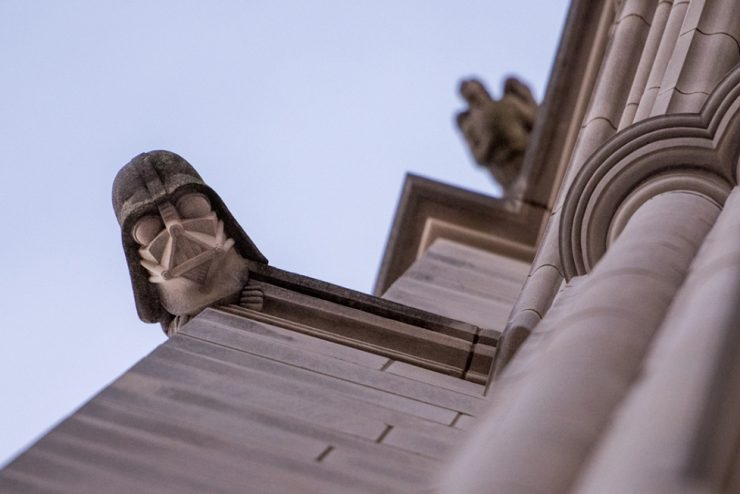This photograph, taken from the unique vantage point of someone standing at the base of a 19th-century-style stone building, captures an upward perspective that accentuates the architectural features. Dominating the left side and center of the image is a striking, concrete statue of the iconic Star Wars character Darth Vader. Unlike the typical black mask, this rendition features a gray face mask, while the helmet retains its traditional dark color, creating a blend of familiarity and surrealism. The stone surface of the building, constructed with gray pillars, extends upward and forms the backdrop. On the right side of the photograph, a partially visible gray column rises, leading the eye to a slightly out-of-focus statue of a stone angel with wings perched on the building's edge. The light blue sky above provides a calm contrast to the structured stonework below, emphasizing the surreal juxtaposition of historical architecture with modern pop culture iconography.